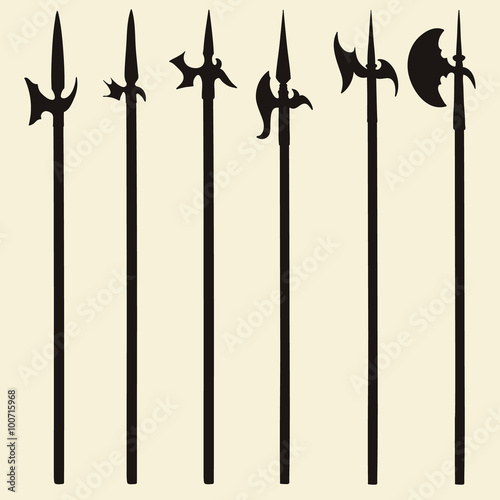The image depicts a collection of six vertical, black silhouettes of medieval battle weapons against a beige or light tan background. These weapons, primarily resembling spears and halberds, are characterized by long, thin poles with sharp, pointy spikes at the top. On either side of these weapons are additional blades of various shapes, including hooks, curved edges, and axe-like blades, designed to inflict maximum damage during combat. The weapons are arranged in a roughly square format, standing tall as if forming a barrier or a fence. The image, which appears to have a digitized or illustrated style, includes some sideways text along the bottom left that reads "Adobe Stock number 100715968," indicating its origin from the Adobe Stock website. The overall scene gives a sense of historical warfare, evoking the brutal and efficient design of medieval armaments.